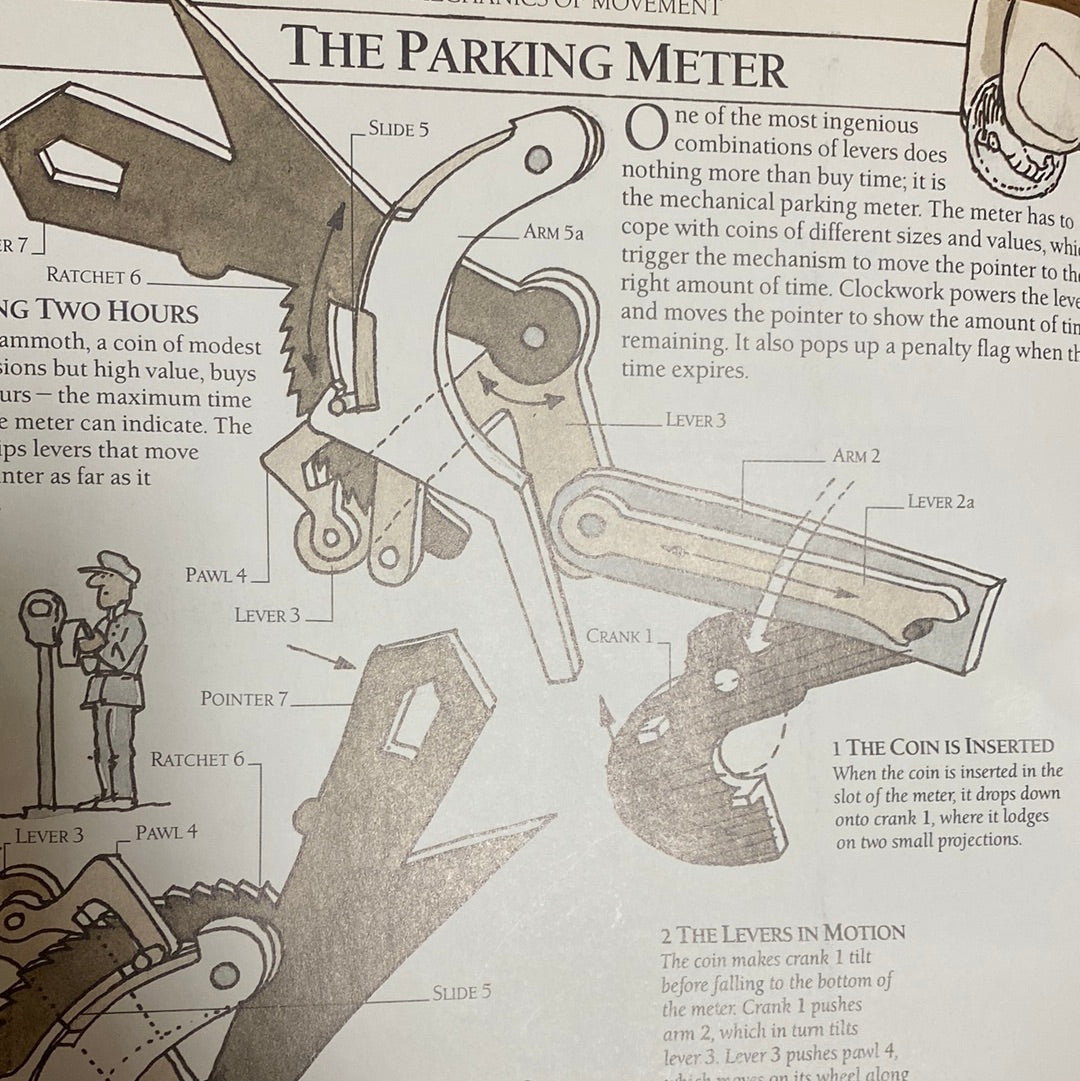The image is a detailed black-and-white diagram from an educational publication, titled "The Parking Meter." It meticulously illustrates the internal workings of a mechanical parking meter, highlighting its ingenious combination of levers and clockwork mechanics designed to buy time. The diagram, accompanied by a labeled illustration, provides a comprehensive look at the parts and their functions: starting with the coin insertion into the slot, it shows how the coin drops onto crank 1, tilting it before the coin falls to the bottom of the meter. This action sequentially moves arm 2, tilts lever 3, and engages pawl 4. The clockwork-powered levers then move the pointer to display the remaining time and pop up a penalty flag when time expires. Additionally, the image includes a cartoonish line drawing of a meter reader writing a ticket and another depiction of the meter's exterior. The entire presentation, rendered in shades suggesting an old-fashioned, pencil-drawn style, serves as an educational resource on the mechanical operation of traditional parking meters.